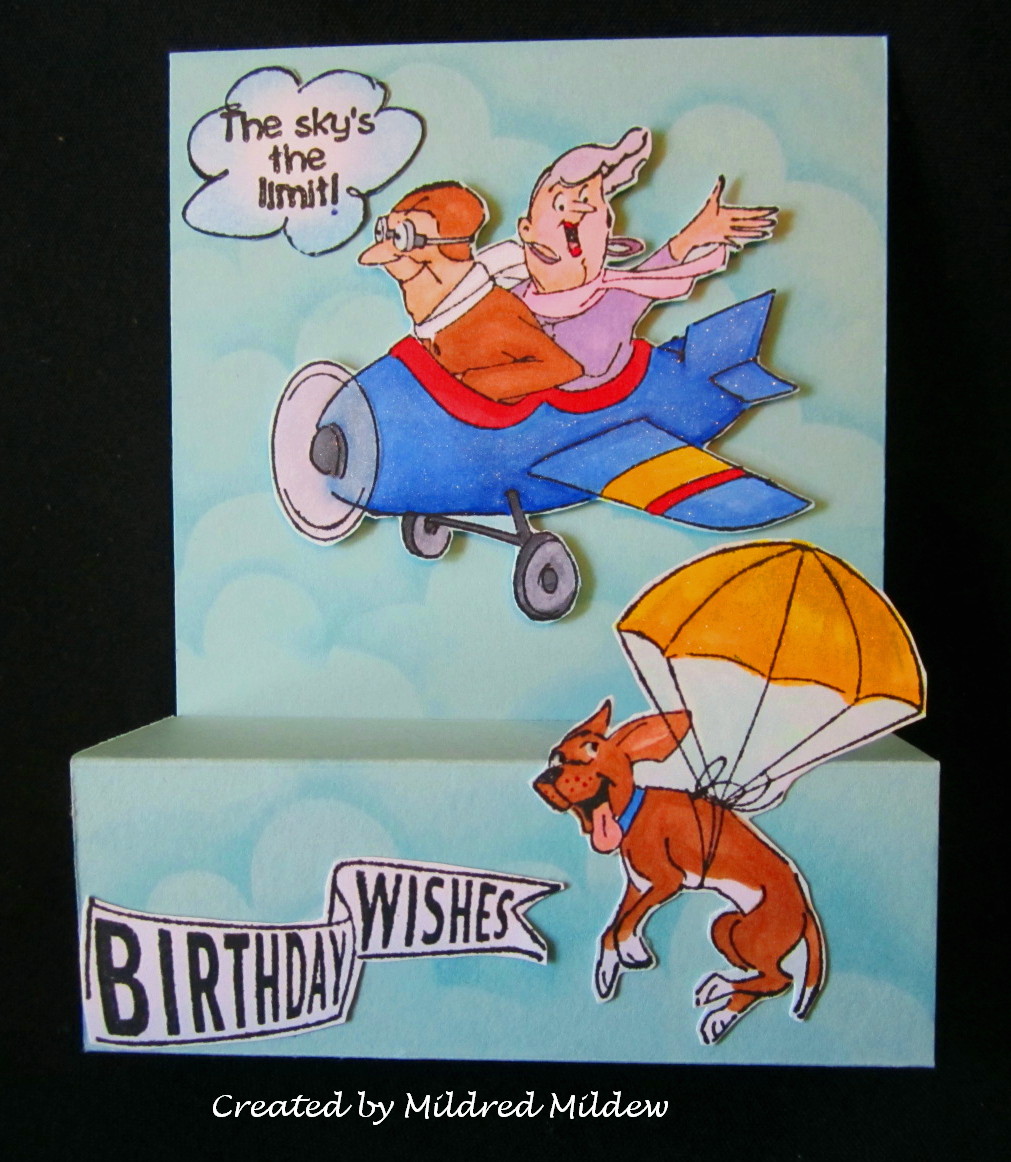The image is a playful and animated depiction, reminiscent of a pop-up birthday card, set against a black background. At its center, a small, cartoon-style blue airplane soars through a light blue sky patterned with fluffy white clouds. Inside the plane, an old man and an old woman are seated, both smiling and seemingly enjoying the flight. The man, dressed in a brown hat, aviator goggles, a brown jacket, and a white scarf, is at the front, focused ahead. The woman behind him sports a purple shirt, white hair, earrings, red lipstick, and a flowing white scarf, with one arm thrown back and a joyful expression on her face. Above the man’s head, a text bubble reads, "The sky is the limit."

Below the plane, a happy brown dog with its tongue playfully sticking out is seen wearing a blue collar and securely attached to a yellow parachute. To the left of the cheerful dog, a ribbon in classic banner style bears the message "Birthday wishes" in black lettering on a white background. The entire whimsical scene is framed by the stark contrast of the pure black background, and beneath the main image, white text elegantly states, “Created by Mildred Mildew.”